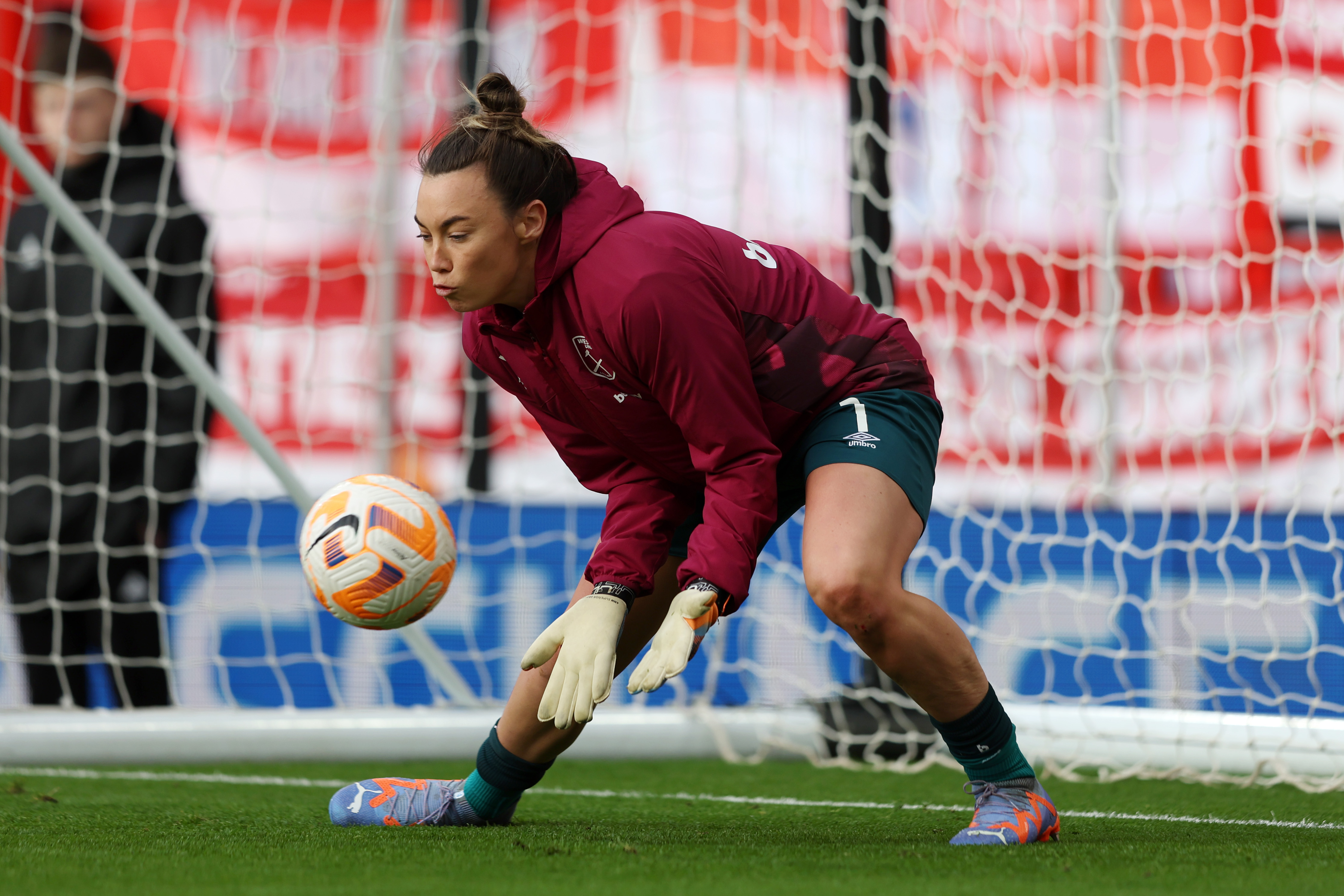The image is an outdoor sports action photograph captured on a sunny day at a soccer field. In the foreground, there's a female goalkeeper of either African or Hispanic descent with tanned brown skin and dark curly hair tied up in a bun. She is dressed in a maroon-red hooded sweater with some white text visible across the back, blue shorts, and black socks. The player is equipped with purple and orange Puma cleats and goalie gloves. She is bent at the waist and knees, crouching in front of the goal net, ready to block an incoming soccer ball, which is white with orange and purple markings and appears to be a Nike ball. The soccer field is lush with green grass marked by white lines. Blurred in the background on the left side of the image, a man dressed in black stands near a marketing banner with red, blue, and white colors behind the goal net. The banner features bold white text, though it's too blurred to read clearly.